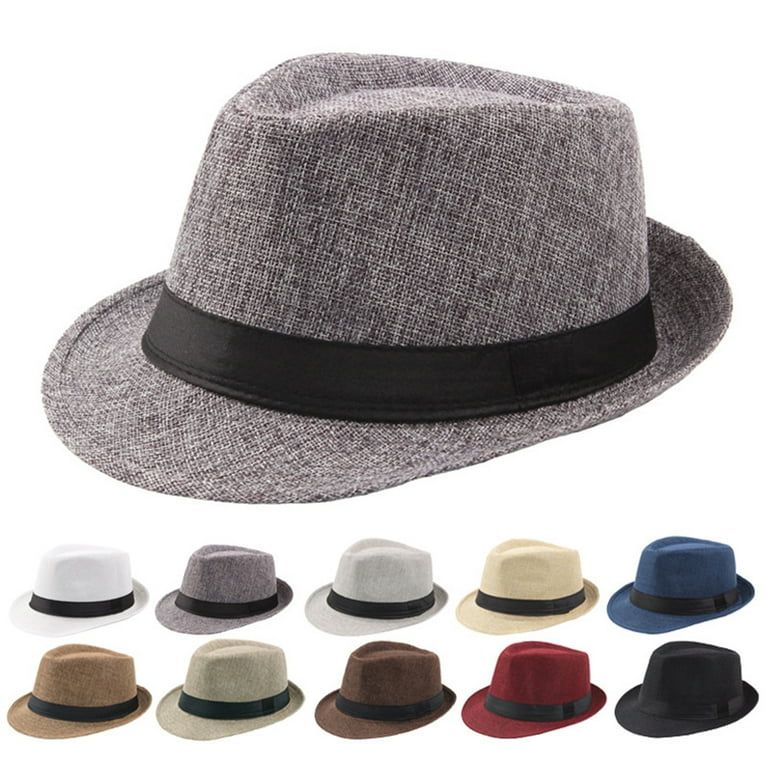The image, resembling a manufacturer's or an e-commerce listing, prominently features a fedora-style hat made of a grayish felt material with a bright black ribbon encircling its base. This hat, characterized by its short brim and tweed canvas appearance, has a slight red tint to its gray hue. Arranged below the main fedora are two rows of five edited versions showcasing an array of colors: white, light gray, light yellow, blue, brown, dark brown, red, and black. Each variation retains the same design with the signature black ribbon, providing a comprehensive display of this stylish hat in multiple hues.